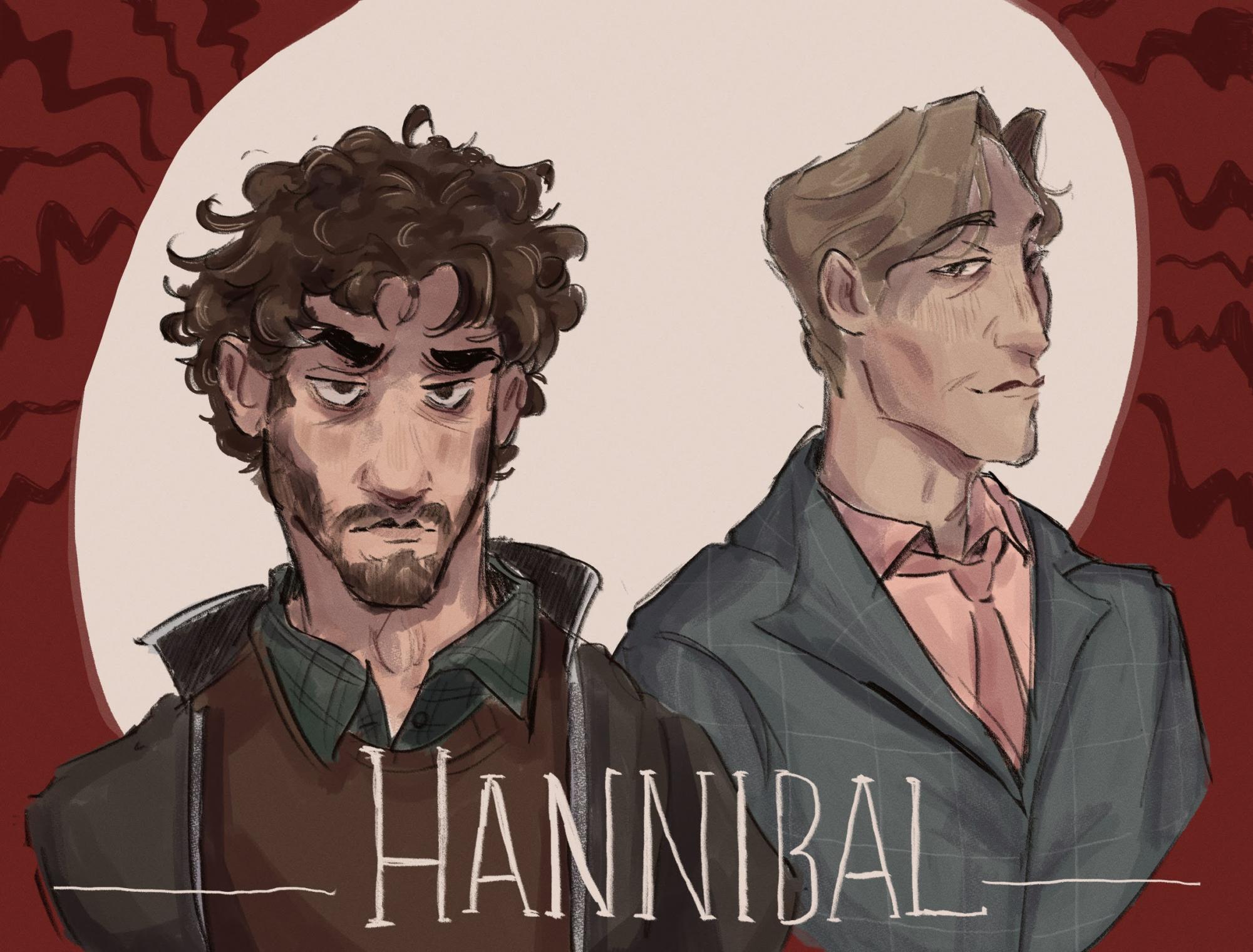The image is a square, hand-drawn artwork with a dark red background accented by squiggly, almost brown lines. Dominating the center is a white circle highlighting two men from the shoulders up, with the text "Hannibal" in white block letters written across their clothing. The man on the left has scruffy, dark brown-reddish hair and a disheveled, somewhat shifty appearance. He is frowning, with a short goatee, arched eyebrows, and is dressed in a layered outfit consisting of a green button-up shirt, a brown sweater, and a dark, possibly black coat. The man on the right has light brown to blonde hair, chiseled features, and a smarmy expression. He gazes to the right while wearing a salmon-colored dress shirt, a slightly darker salmon tie loosely pulled apart at the neckline, and a dark gray or slate blue suit jacket. Both men are depicted mid-torso up, with no arms visible.